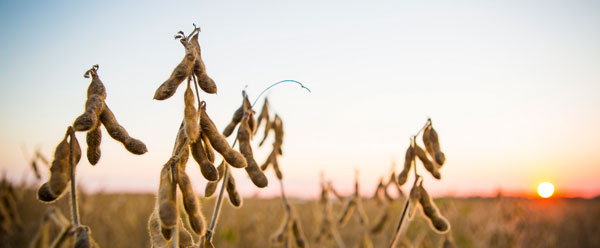The photograph captures a serene outdoor scene at sunset. The sun, a glowing white orb, is positioned near the bottom right of the image, emitting a warm orange light that bathes the horizon. The sky transitions from a light blue in the top left corner to a hazy white, enhancing the dreamy ambiance. In the foreground, the focus is on a cluster of tan, fuzzy pods hanging from stems that curve downwards, resembling some variety of wheat or cattails. These stalks stand out sharply against the blurred background of a vast field stretching to the horizon, completing the tranquil landscape.